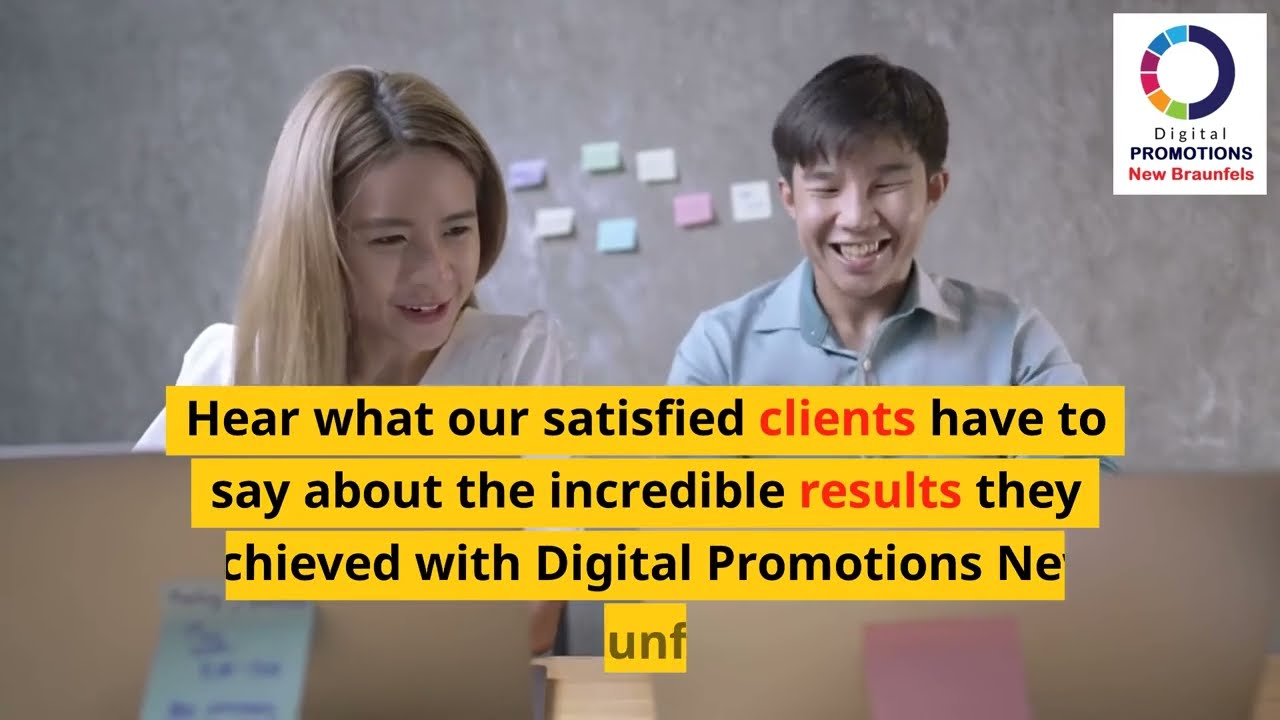The image features a young girl and a young boy, both appearing to be around 14 to 15 years old, sitting side by side at a desk with computers. The girl, on the left, has long, light brown hair and is wearing a white blouse. The boy, seated to her right, has dark hair and is dressed in a light blue button-down collared shirt. They are both of Asian descent and are smiling and laughing at something displayed on the boy's computer screen. The background showcases a gray wall adorned with sticky notes in various colors—purple, green, yellow, and pink—positioned between their heads. Overlaying this scene, text in black partially reads: "Hear what our satisfied clients have to say about the incredible results they achieved with digital promotions, UNFs." Additionally, the upper right-hand corner of the image includes a white square with a circular logo split into navy blue and rainbow colors, accompanied by the text “Digital Promotions” in black and “New Braunfels” in red.